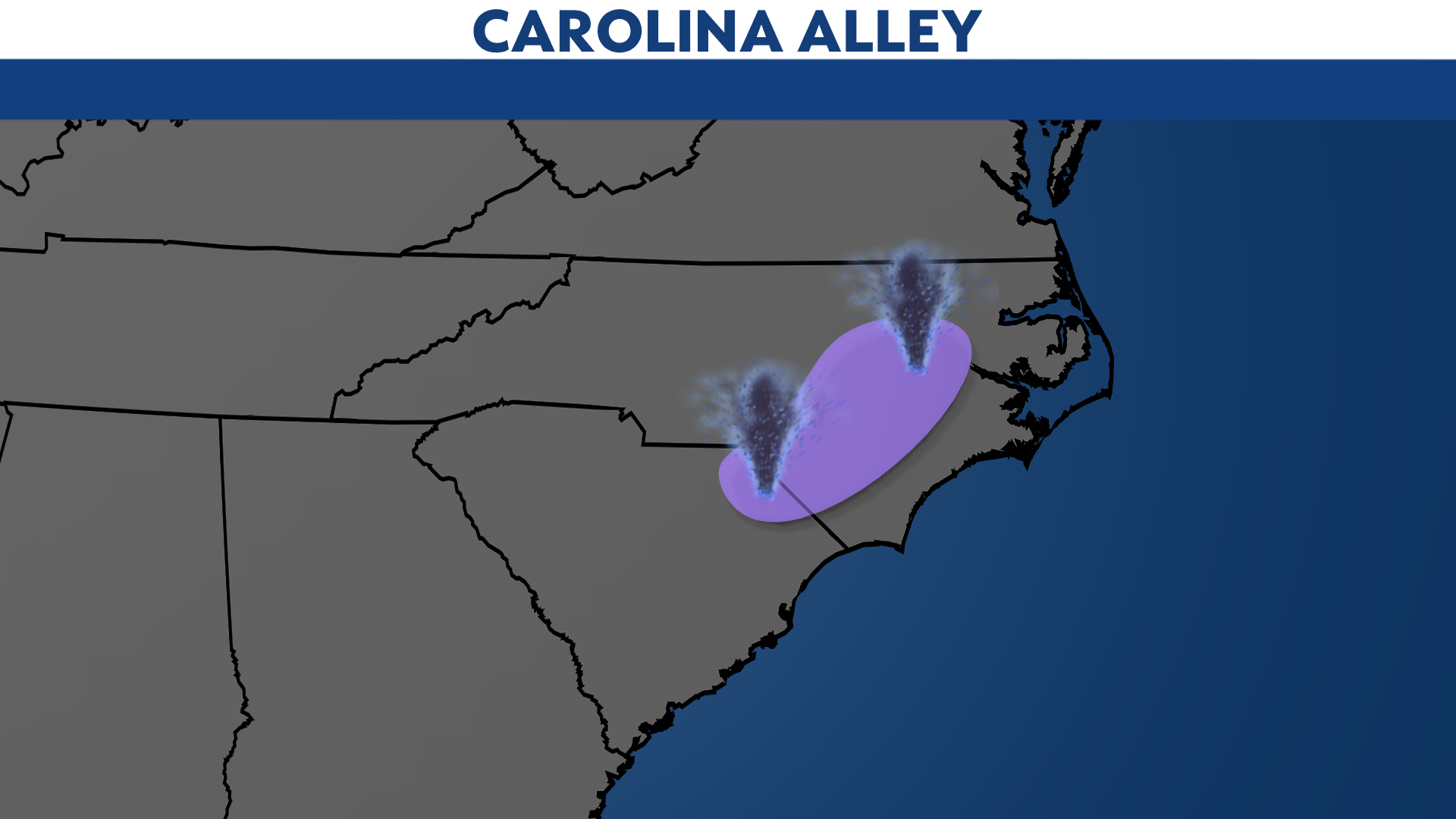The image, likely an illustration from a weather map, prominently displays the title "CAROLINA ALLEY" in bold, all-capital letters at the top in blue, matching the color of the surrounding sea depicted on the right side of the map. This smooth, solid blue backdrop indicates it is the ocean adjacent to the southern United States. The map features Virginia at the top and Georgia at the bottom, with a specific focus on North Carolina, though the states are not labeled and rendered in gray. Centered over North Carolina and extending slightly into South Carolina, a large purple oblong shape dominates the map, within which two tornado icons are positioned at opposite ends. This visual representation highlights an area known as Carolina Alley, indicating a region prone to tornado activity akin to Tornado Alley in the Midwest.